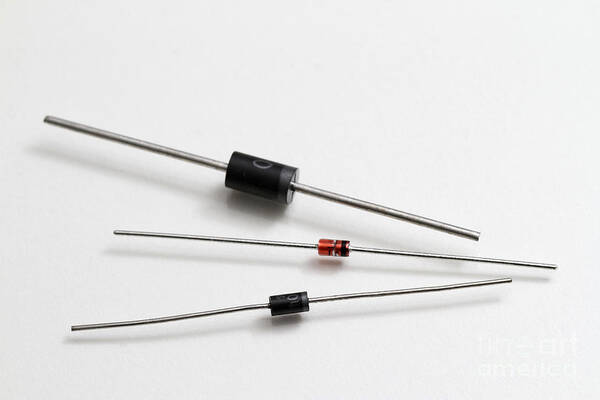The image shows three slender metal components horizontally aligned on a white background, each varying in thickness and featuring cylindrical connectors in their middles. The top component, the thickest of the three, possesses a black plastic cylinder with possible text on it, hinting at an electronic or electrical purpose. The middle component, the thinnest, has a red cylinder with a black band, possibly resembling a resistor. The bottom component, intermediate in thickness, features a black cylinder similar to the top one, but smaller. Shadows cast by the components add depth to the otherwise stark, white background.